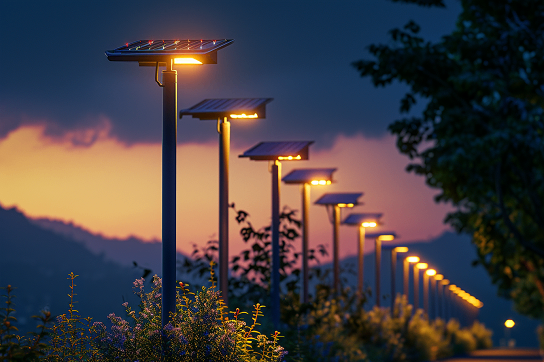The image is a detailed close-up of a row of solar-powered streetlights taken at dusk, just before sunset. The solar panels are prominently facing towards the viewer, with orange lights illuminating the poles underneath each panel. The scene captures around 15 to 20 streetlights aligned diagonally from the front left to the back right, creating a perspective that showcases their number and distance.

In the background, the sky exhibits a rich orange hue with scattered clouds, typical of the moments just before the sun fully sets. The shadowy outlines of mountains add depth to the horizon, and a hint of twilight remains in the sky, emphasizing the time of day. The landscape includes some shrubs and greenery that run parallel to the row of streetlights, adding a touch of natural scenery. Additionally, a few plants with partially visible green leaves and possibly purple or pink petals are discernible in the foreground. To the right, there are visible branches and green leaves of a tree, though the full tree is not captured in the frame. The image effectively combines the elements of renewable energy, natural beauty, and the tranquil transition from day to night.